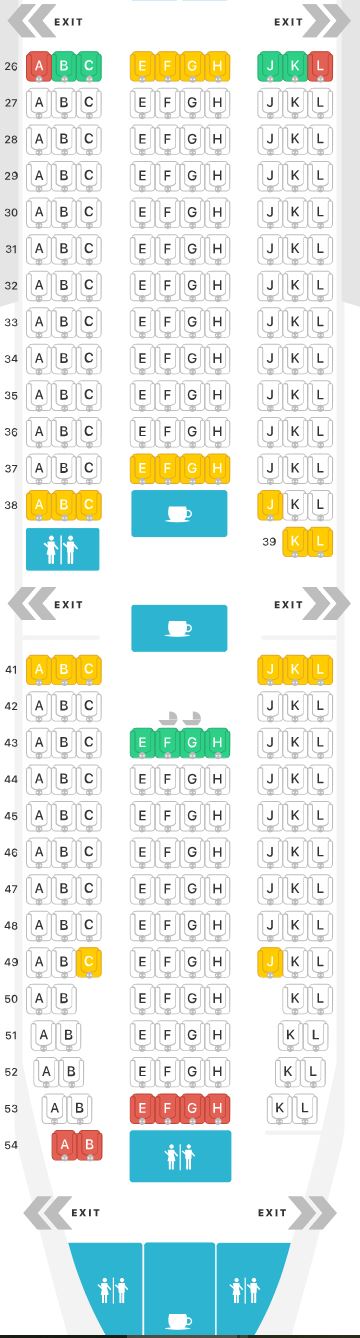This image appears to be a detailed seating chart or layout, possibly for an auditorium, theater, or similar venue. The background is predominantly white, with gray areas on both the left and right sides. 

On the left side starting from the top and moving downward, there are numbers listed vertically: 26, 27, 28, 29, 30, 31, 32, skipping to 38. Next to each of these numbers, there are letters: A, B, and C, in various colors. For instance, row 26 features a red 'A,' green 'B,' and green 'C.' The middle block of these rows (EFGH) features mostly yellow, while 'J' and 'K' are green and 'L' is either white or red in the 26th row. In the 37th row, the middle block is yellow, and row 38's ABC section is yellow as well, with the middle section depicted by a blue rectangle containing a white cup icon. 

Moving further down, there’s a woman and man icon in a rectangular block, indicating restrooms. Row 39 has a yellow 'K' and 'L,' followed by another blue rectangle with a white cup icon. 

The numbers then continue from 41 to 54 on the right side. Row 41 includes yellow letters for ABC and JKL, while EFGH is colored green for row 43. Row 49's EFGH section is in red. Row 53's A and B are colored red. Row 54 does not have middle or right side numbers but includes a blue tab with a woman and man icon.

Throughout the layout, there are “Exit” signs marked by double greater-than symbols (>>) on the left and double less-than symbols (<<) on the right, strategically placed for easy visibility.

This detailed seating chart or layout indicates various sections and areas, complete with color-coded seating, amenities, and exits for clear navigation.